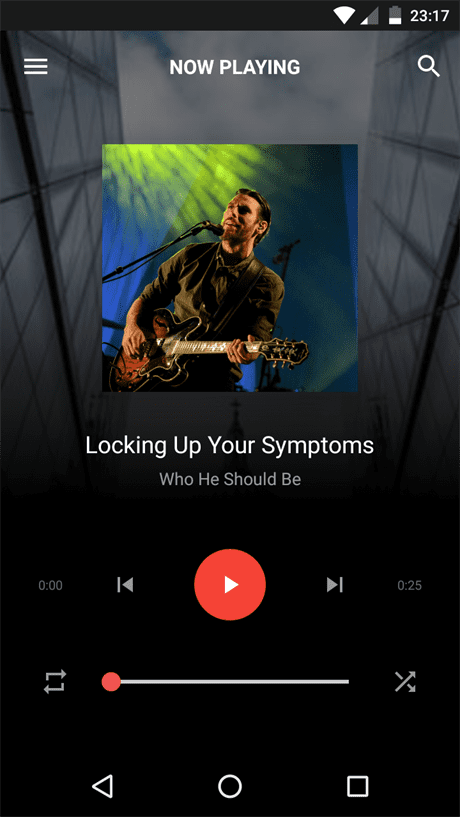The image is a vertically rectangular screenshot taken from a cell phone, depicting a music app interface. At the top, a thin black horizontal banner displays the Wi-Fi signal bars, battery icon, and the time "23:17" on the right side. Below the banner, the interface features the app's control elements, starting with the menu icon—three horizontal bars—on the left, the text "NOW PLAYING" in all caps at the center, and a search icon on the right.

Centered below these elements is an image of a man with a microphone playing an electric guitar. Directly beneath the image is the song title "Locking Up Your Symptoms" and the artist's name "Who He Should Be."

The central feature of the interface is a large red play button flanked by back and forward buttons on its left and right sides, respectively. The total duration displayed is "25 seconds." Below the play button is a progress slide bar, currently set at "0:00." The slide bar is bookended by the repeat icon on its left and the shuffle icon on its right.